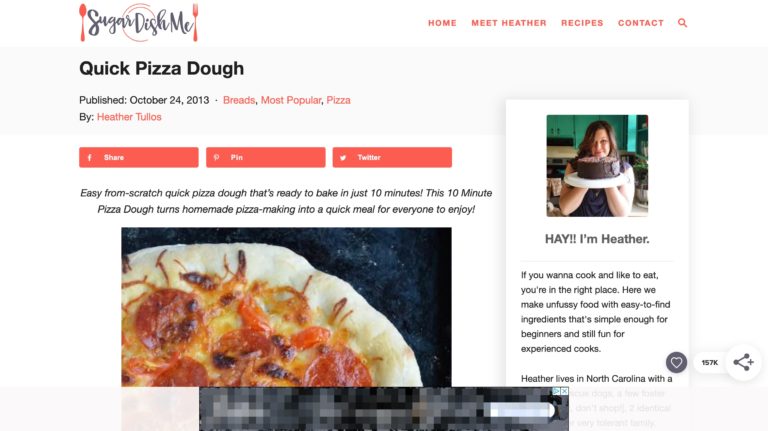The image is a snapshot from the "Sugar Dish Me" website, resembling a charming mommy blog with various culinary delights. On the right side of the site, there is a welcoming image of a woman named Heather, who is the blog's author. Next to her picture, a friendly greeting reads, "Hey, I'm Heather. If you want to cook and like to eat, you're in the right place. Here we make unfussy food with easy-to-find ingredients that are fun for beginners and still enjoyable for experienced cooks."

The website features a soothing color palette with soft whites and warm orangey reds, enhancing its inviting atmosphere. In Heather's photo, she proudly holds up a luscious chocolate cake, embodying the blog's theme of delightful home-cooked meals. 

The main focus of the page is a highlighted recipe for "Quick Pizza Dough," published on October 24, 2013. The recipe promises an easy, from-scratch pizza dough that is ready to bake in just 10 minutes, making homemade pizza an accessible and quick meal for everyone to enjoy. Accompanying this is a mouth-watering image of a pepperoni pizza with light, soft dough, visually underscoring the recipe's simplicity and appeal.

At the bottom of the page, a blurred-out banner ad is visible, while the top left corner proudly displays the whimsical "Sugar Dish Me" logo. The logo features cute cursive writing with a small dish in the middle, flanked by a fork and spoon on either side, perfectly encapsulating the blog’s charming and approachable vibe.